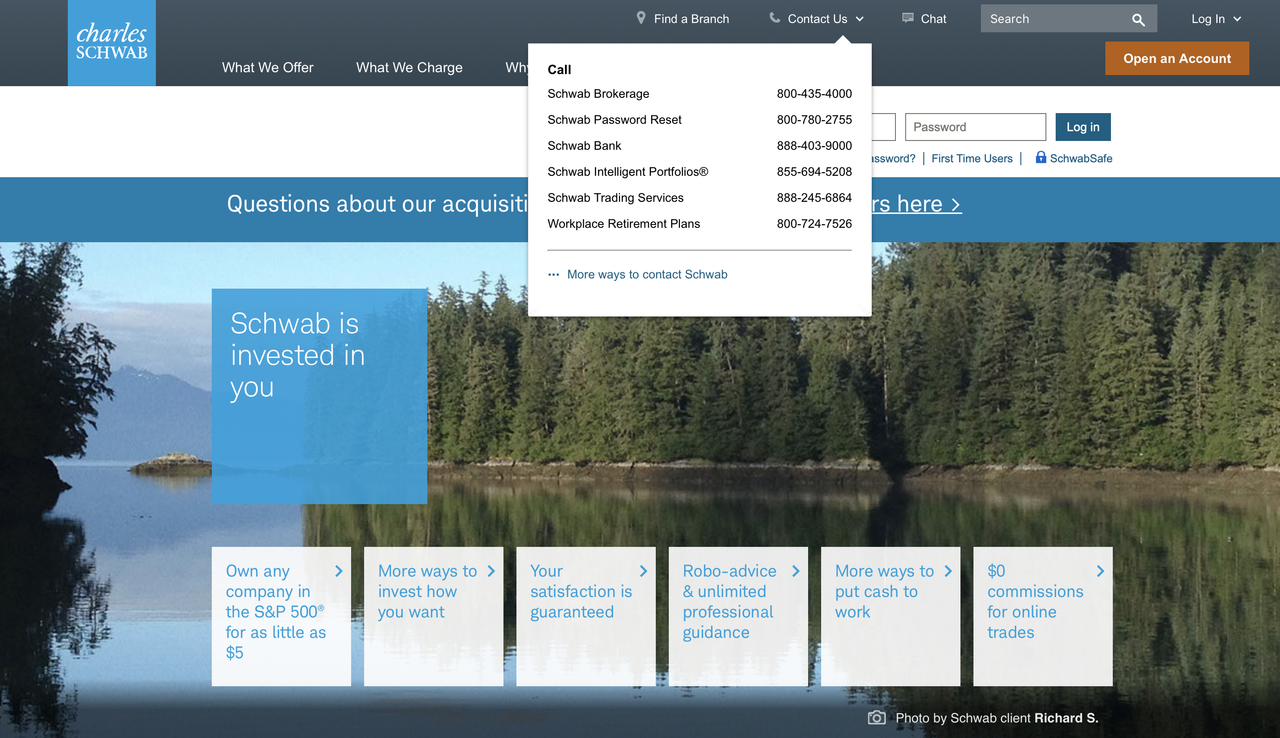The top of the webpage features a gray bar, approximately an inch thick, stretching across the entire width. On the left side of this bar, there's a small blue box with white text reading "Charles" on the top and "Schwab" beneath it. To the right of this blue box, the gray bar contains white text stating, "What We Offer," "What We Charge," and partially obscured by a white drop-down box, "WH." 

Inside the drop-down box, written in black, is a list of contact options:

- "Call Schwab Brokerage," followed by "800-435-4000"
- "Schwab Password Reset," followed by "800-780-2755"
- "Schwab Bank," followed by "888-403-9000"
- "Schwab Intelligent Portfolios," followed by "855-594-5209"
- "Schwab Trading Services," followed by "888-245-6864"
- "Workplace Retirement Plans," followed by "800-724-7528"

At the bottom of the drop-down box, in blue text, it reads "More Ways to Contact Schwab."

Above this drop-down box, still within the gray bar, is a sequence of white icons and text:
- A map pin icon next to "Find a Branch"
- A phone icon next to "Contact Us" with a drop-down arrow (corresponding to the white drop-down box described)
- A chat bubble or voice icon next to "Chat"

To the right of these icons is a gray search bar with "Search" written in white on the left and a white magnifying glass search icon on the right. Further right is white text that reads "Login" with a drop-down arrow.

Below the search bar and login section is a coin bar displaying "Open an Account" in white text.

Adjacent to the search bar and drop-down menu is a white search bar with "Password" written in black inside it. To the right of this is a blue box with white text that says "Login." Below this is a phrase, "Password," emerging from the drop-down box with a question mark, a dash, "First Time Users" in blue, followed by another dash, a blue lock icon, and "SROB Safe" in blue.

Underneath this is another blue bar, about an inch thick, spanning across the page. In the center of this bar, in white, it partially reads "Questions About or Acquisitions" (with "Acquisitions" partially hidden by the drop-down menu). To the right of the drop-down menu, a white arrow points left with the word "Here."

Below this blue bar is an image of a lake flanked by pine trees on both sides and mountains in the background. In the center-left of this lake image is a blue box with white text stating, "SROB is investing in you."

Below this text are six small white boxes with blue writing:
1. "Own Any Company in the S&P 500 for as little as $5"
2. "More Ways to Invest How You Want"
3. "Your Satisfaction is Guaranteed"
4. "Robo-Advice and Unlimited Professional Guidance"
5. "More Ways to Put Cash to Work"
6. "Zero Dollar Commissions for Online Trades"

Near the bottom right of the lake image, slightly centered, is a small white camera icon with the text "Photo by SROB Client Richard S."